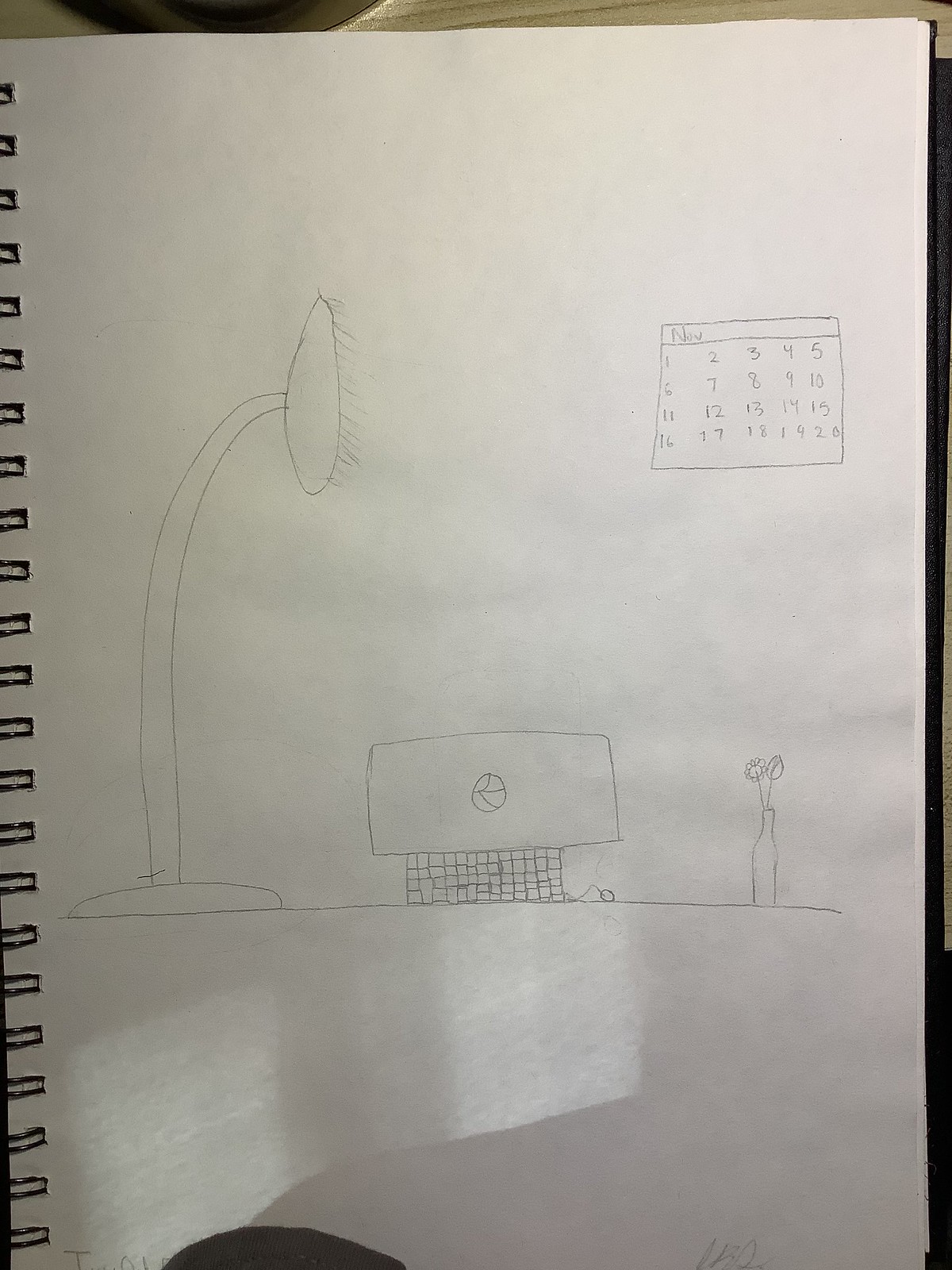The image captures a detailed drawing on the right-hand page of a white, spiral-bound sketchbook, with the black spirals visible along the left side. The background hints at a tabletop where the sketchbook is placed. The main elements of the drawing include a fan or light fixture on the left, a flat line representing a table surface, and a chair tucked under the table. To the right, there's a computer monitor with a keyboard in front of it, and a vase housing two flowers — one resembling a sunflower and the other an underdeveloped rose. Above the vase, on the wall, hangs a calendar labeled "NOV" for November, numbered from 1 to 20. There is also lettering near the bottom of the page, below the table line, alongside a small indistinguishable black area. The meticulous sketch is rendered in pencil, detailing the scene with precision.